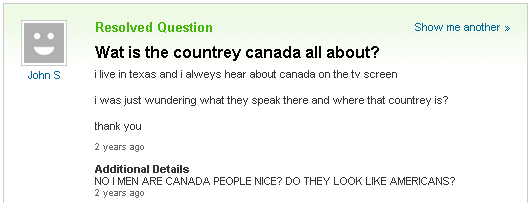A horizontal image showcasing a partial view of a webpage, accessible from either a computer or smart device. The image is bordered by a thin black line on the top, left, and right sides, with the bottom edge blending into the white of the computer screen. In the upper left-hand corner, there is a box with a smiley face icon, beneath which the name "John S." is displayed in blue text. Below this, "resolved question" is written in green.

On the upper right-hand side, in blue text, there is an option labeled "show me another," which appears clickable. Beneath the "resolved question" label, a poorly typed inquiry appears with misspelled words and improper capitalization: "what is the country Canada all about?" This is followed by a user message stating, "I live in Texas and I always hear about Canada on the TV screen. I was just wondering what they speak there and where that country is. Thank you," noting that the question was posted two years ago, with multiple spelling errors throughout the text.

Further down, "additional comments" is written in bold black text, beneath which an emphatic query reads, "NO, I MEAN, ARE CANADA PEOPLE NICE? DO THEY LOOK LIKE AMERICANS?" Also marked as being posted two years ago.